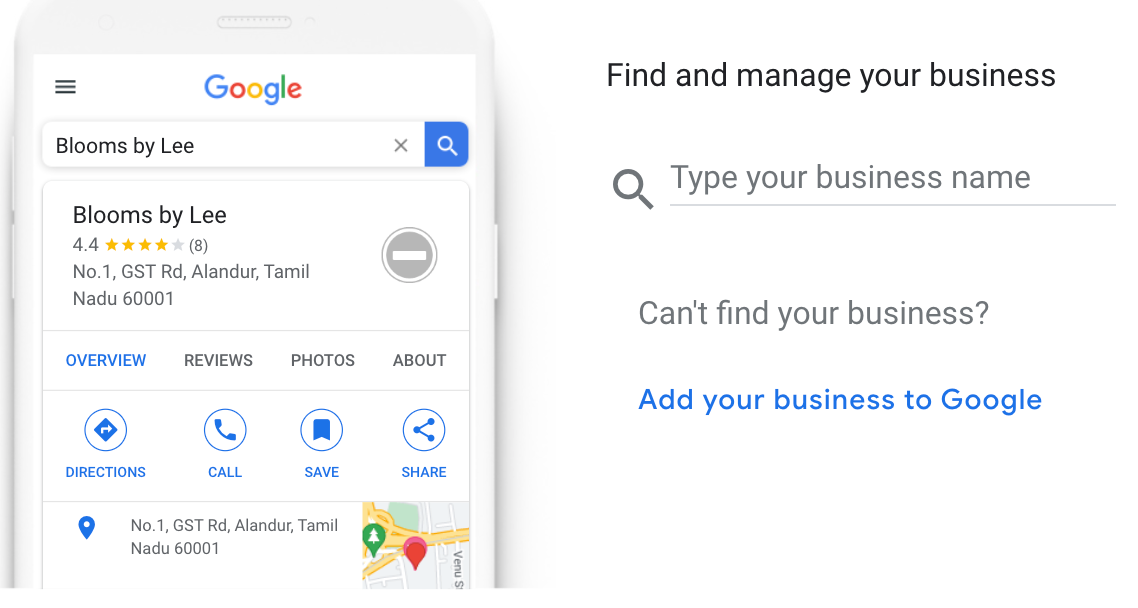The photograph showcases the upper part of a smartphone screen displaying a Google search result for "Blooms by Leah." On the top left corner of the screen, the familiar three horizontal lines icon, which accesses the menu, is visible. Centered prominently is the Google logo with a search field just below it. The search query "Blooms by Leah" is entered into this field, flanked on the right by an 'X' to clear the query and a blue magnifying glass icon to initiate the search.

Directly below the search field, the search result for "Blooms by Leah" appears, featuring the business name along with a rating indicated by four gold stars followed by the number eight in parentheses, showing that it has been reviewed by eight people. Beneath the business name, the address "Number 1, GST Road, Alandur, Tamil" is listed, followed by "New Madu, 60001." To the right of the address, there's a gray circle containing a white horizontal line, reminiscent of a minus sign.

Further down are four tab options: "Overview," "Reviews," "Photos," and "About." The "Overview" tab is highlighted in blue, indicating it is currently selected. Below these tabs, there are four functional buttons labeled "Directions," "Call," "Save," and "Share."

On the right side of the screen, there is a section titled "Find and Manage Your Business." Within this section, a search field prompts the user to type their business name, indicated by placeholder text in gray font. To the left of the search field, there is a small magnifying glass icon. Below this, the text "Can't Find Your Business?" appears in gray, followed by a blue link reading "Add Your Business to Google."